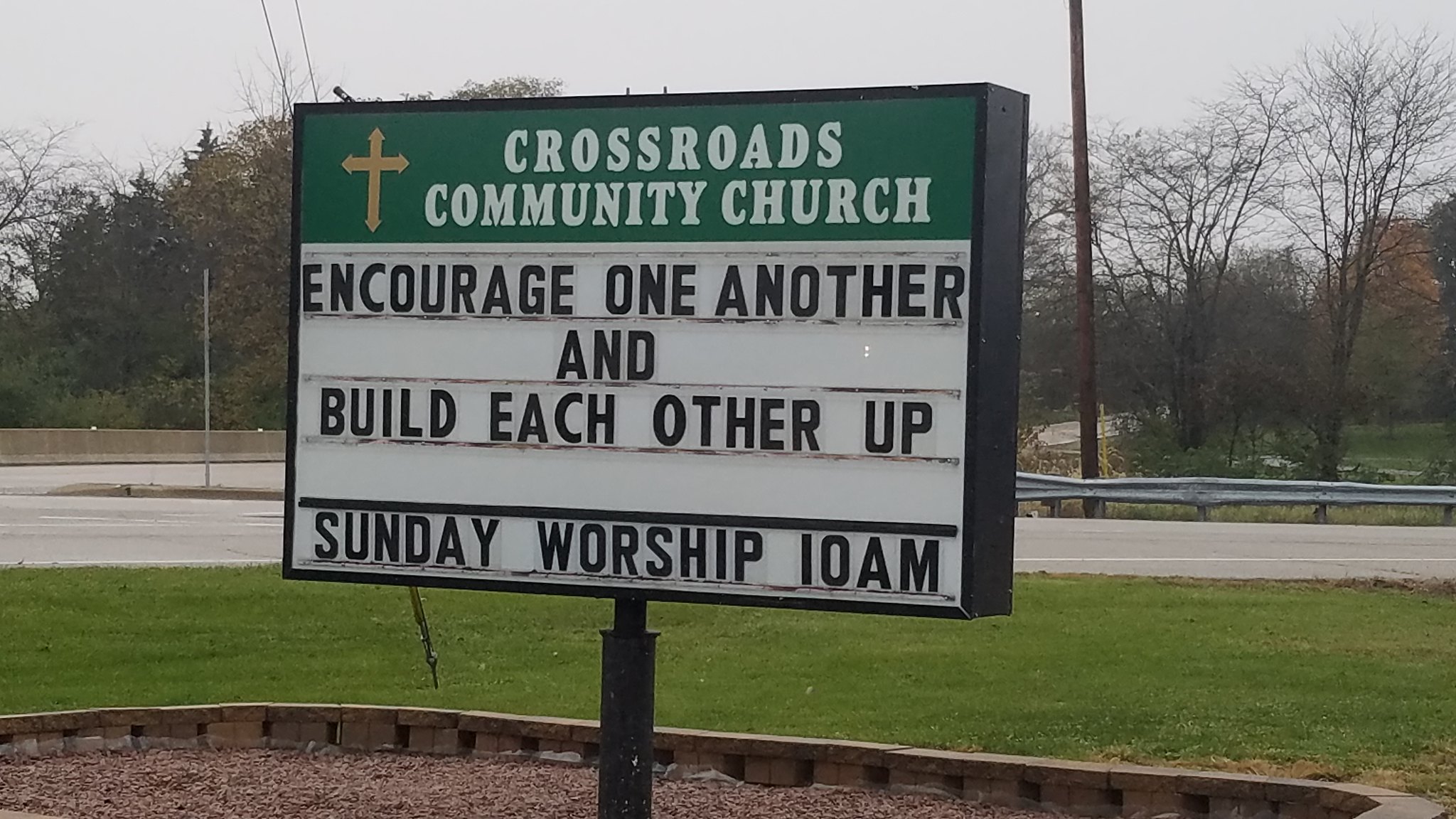The image features a green and white marquee sign for Crossroads Community Church. The top portion of the sign is green, adorned with a gold cross to the left and the text "Crossroads Community Church" in white lettering to the right. Below this, on a white background with black text, the sign reads "Encourage One Another and Build Each Other Up" and "Sunday Worship 10 a.m." All the text is capitalized. The sign is mounted on a black pole and set within a mulched area bordered by cement blocks. This area is surrounded by a broad expanse of green grass. Beyond the grass, there is a road with a silver guardrail and a curb, leading to a parking lot. The background features a line of trees, and the sky above is overcast and filled with clouds, creating a white, gloomy atmosphere.